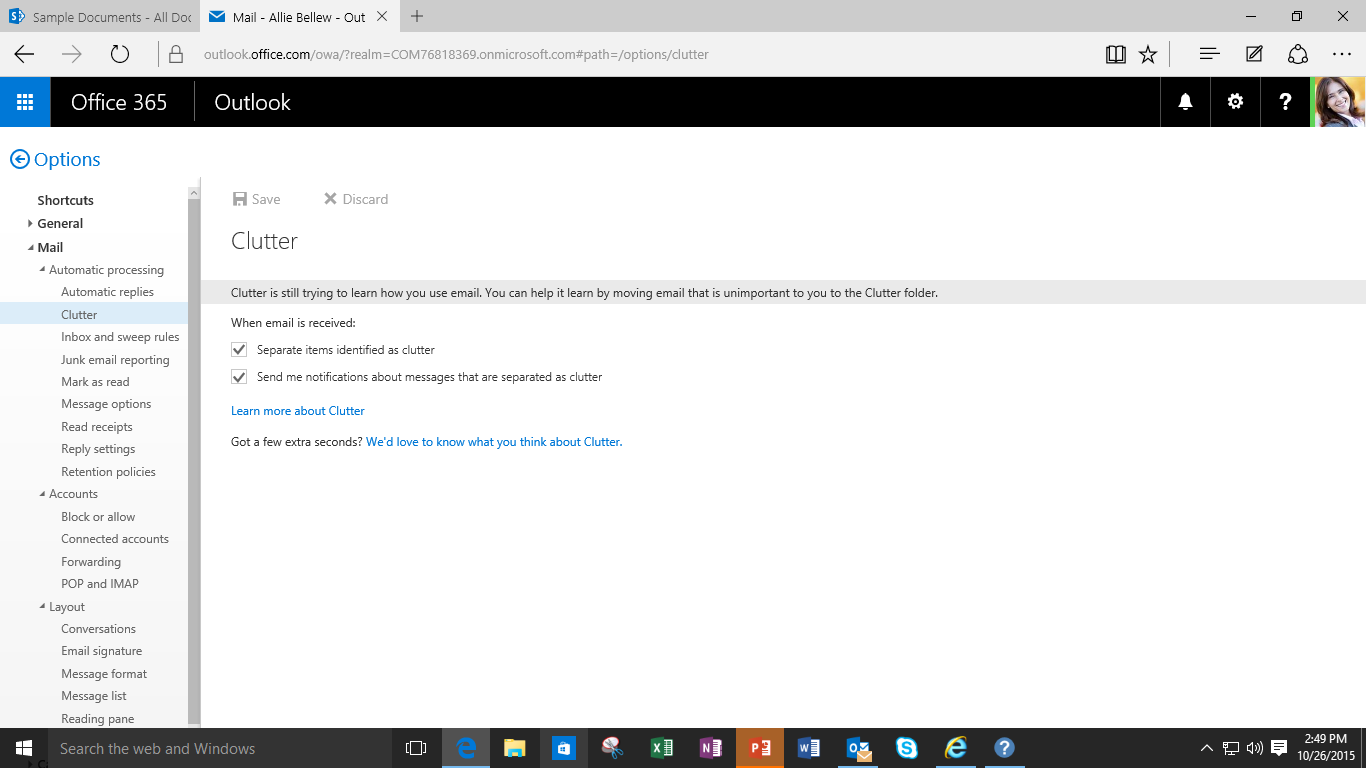The image appears to be a screenshot of a typical Office 365 web interface. On the left side of the screen, there are several blue icons, and prominently displayed text reads "Office 365" alongside "Outlook." Below that, the URL "outlookoffice.com" is visible. This screen seems to show a sample document and email interface with options for managing mail.

To the left, a vertical navigation bar features various shortcut options such as "General" and "Mail," each with sub-categories like "Automatic Replies," "Inbox," "Sweep," "Junk Email," "Options," "Read Receipts," "Reply," and "Accounts." These categories help in navigating through the email settings.

On the right-hand side, there are sections titled "Clutter" and other organizational tools. At the very bottom of the screen, several desktop shortcut icons are visible, including Internet Explorer, Excel, PowerPoint, and Mail, among other standard icons that commonly appear on a user's desktop environment.

In the top right corner, there's a profile picture of the user, along with the current time and date. The image gives a snapshot of a common situation where someone is multitasking between managing their emails and accessing various Office 365 applications while also browsing the web.